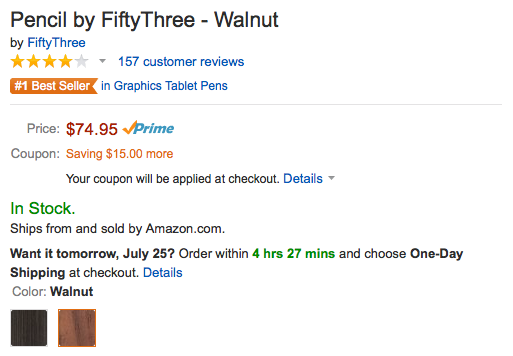A detailed description of the image, cleaned up and organized:

---

The image showcases a portion of an Amazon listing, set against a completely white background. At the top, in black text, it reads "Pencil by 53 - Walnut." Directly underneath, in blue text, it states "by FiftyThree." The product has a rating of four out of five stars, based on 157 customer reviews. Highlighting its popularity, there is an orange banner with white text declaring it the "Number 1 Best Seller in Graphic Tablet Pens."

Below this banner, a thin gray line separates the header from the price information. The product is priced at $74.95 and features a Prime checkmark. Additionally, a note mentions that you can save $15 or more with a coupon that will be applied at checkout, with a link to more details.

The listing further indicates the product is in stock with green text, followed by the information that it ships from and is sold by Amazon.com. It offers a delivery option to have the item by tomorrow, July 25th, if ordered within four hours and 27 minutes, and by selecting one-day shipping at checkout.

Under the shipping details, the text "Color" is followed by "Walnut" in bold. Two color swatches are displayed: the left square is a very dark brown, and the right square is a more typical brown, outlined in orange.

This listing comprehensively details the "Pencil by 53 - Walnut" product priced at $74.95 on Amazon.